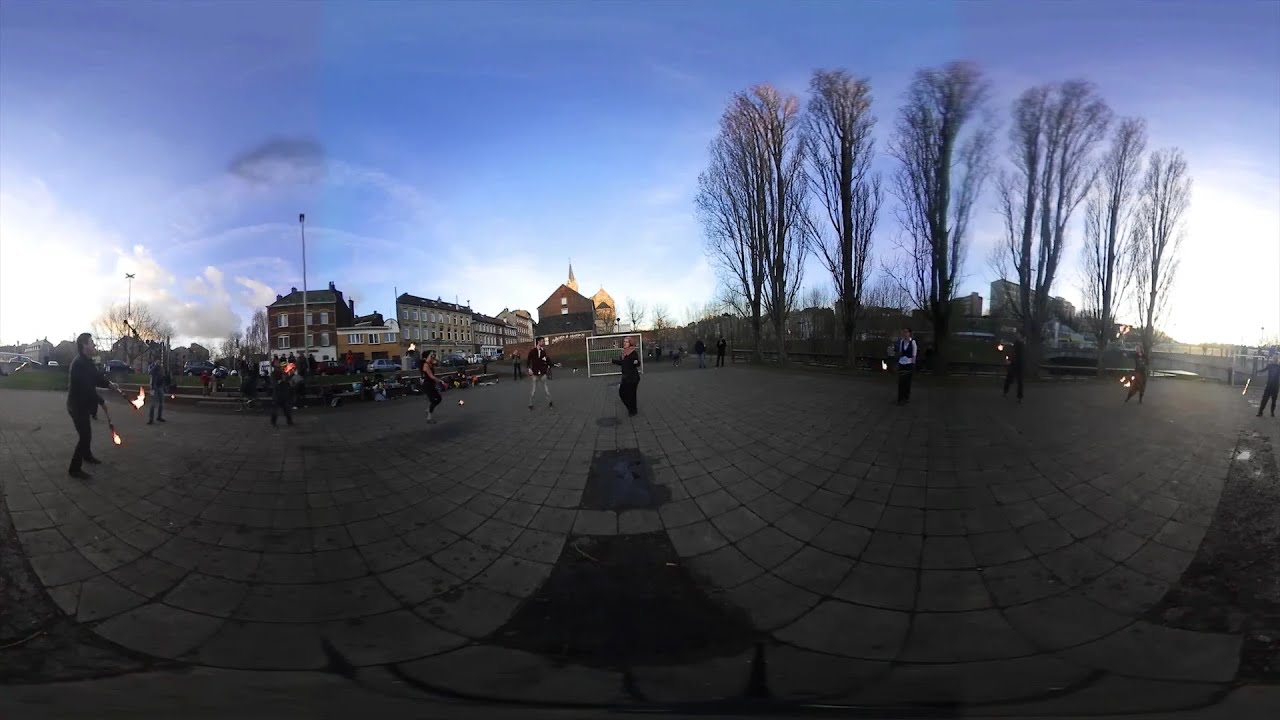This photograph, taken during either early morning or late evening before nightfall, depicts an outdoor scene with a panoramic, fisheye effect that creates a rounded distortion. The ground is laid with gray stone tiles, forming a brick courtyard. In the foreground, several people, mostly dressed in black, are gathered, some seemingly dancing or engaged in a ceremony. They are holding flaming sticks, with one individual on the far left clearly juggling three fiery batons; their hands and the batons are aflame.

The surrounding environment includes a variety of elements: On the back left, partly cloudy sky frames several multi-story buildings that might be apartments or a church. Five or six tall, barren trees, likely indicating a winter setting, stand prominently in the background. Between two distinct dome-shaped sidewalk areas, separated by a dirt patch, people can be seen walking. The main colors in the image are blue, white, and brown. The bright light on the horizon suggests a low sun, enhancing the scene’s dynamic atmosphere with a prominent use of light and shadow.